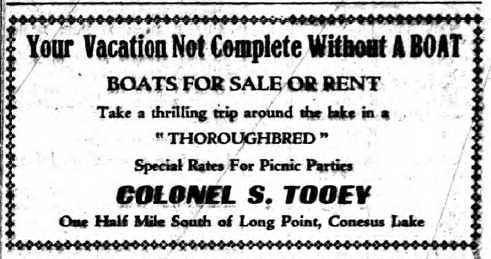This rectangular image, likely an old-fashioned ad clipped from a newspaper or magazine, features a simple, white background bordered by a line of small black dots. Dominating the top of the ad in large, bold black letters, it declares, "YOUR VACATION NOT COMPLETE WITHOUT A BOAT," with the word "BOAT" prominently capitalized. Below this, in slightly smaller all-capital letters, it offers "BOATS FOR SALE OR RENT." Further down, the text encourages viewers to "Take a thrilling trip around the lake in a 'THOROUGHBRED'," with the word "THOROUGHBRED" emphasized in quotations and capitalized. The ad also highlights "Special rates for picnic parties." In a larger bold font, the name "COLONEL S. TOOY" is displayed. Finally, in smaller black text at the bottom, the ad provides a location: "One half mile south of Long Point, Conesus Lake."